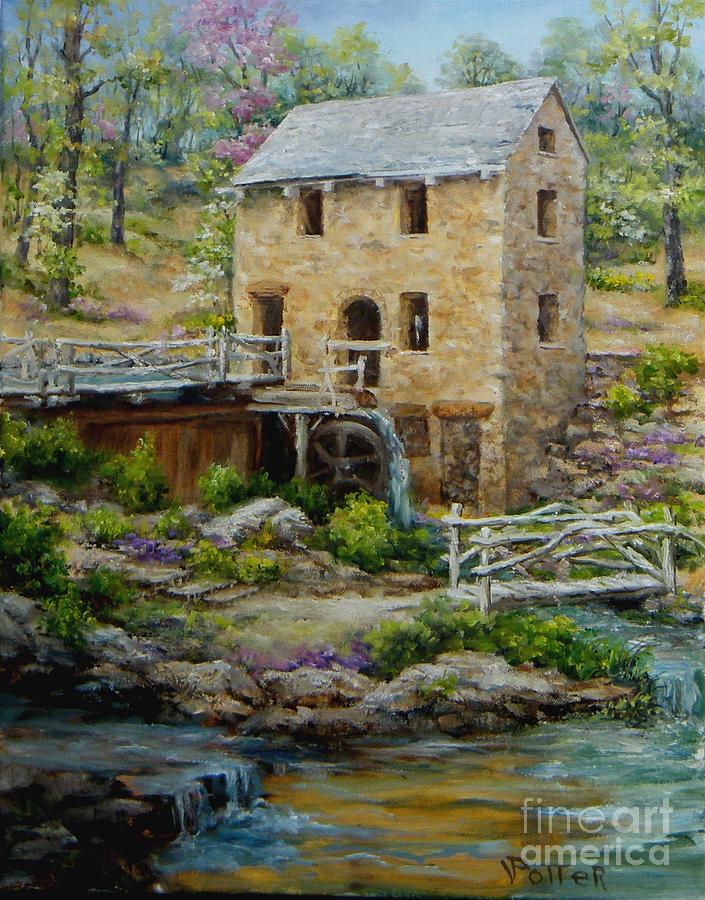This captivating painting, executed in oil by the artist Potter, depicts a quaint and weathered stone mill nestled against a hillside, crowned with a deteriorated gray roof. The mill features multiple open windows that reveal a figure gazing outward. Prominently, a sturdy water wheel channels the stream's flow, which cascades over rocky terraces and creates miniature waterfalls. A rickety wooden split rail railing encloses the top of the dam, adding to the rustic charm. 

In the foreground, a small footbridge spans the stream, inviting pedestrians to cross the serene, blue waters. The banks of the stream are adorned with lush greenery and vibrant purple flowers, possibly violets, creating an idyllic natural setting. Surrounding the mill and stream, the hill is dotted with shrubs and various flowers, while the backdrop of tall trees, some adorned with pink and white blossoms, completes the picturesque scene. A clear blue sky above adds to the tranquility of this composition. The painting carries a watermark, "Fine Art America," emphasizing its place in a collection of esteemed artworks.